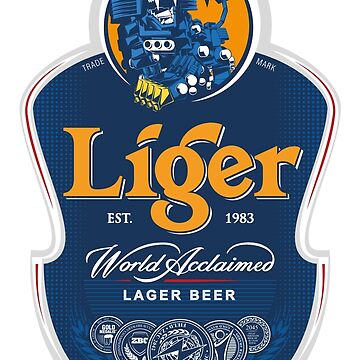The image depicts a detailed beer logo set against a solid white background. The central element of the logo is a large, blue badge-like shape that is partially cut off at both the top and the bottom. The badge has white outlines and features an array of text and designs in orange, gold, and white. 

At the top of the badge, there's a circular design which appears to feature a mechanical, robot-like figure resembling a "Liger" (a fusion of a lion and tiger). The robot has blue and metallic orange features, including boxy, mechanical parts that give it a Transformer-like appearance. Flanking this circular design are the words "Trade" on the left and "Mark" on the right in small white letters.

The name "Liger" is prominently displayed in large, orange letters in the center of the badge. Directly below, in smaller white text, it reads "Est. 1983," followed by "World Acclaimed" written in cursive and underlined in red. Beneath that, it states "Lager Beer" in standard print. The bottom of the badge features overlapping circles that might represent awards or medals the beer has won, adorned with some unreadable white print. The overall design combines elements of modern robotics with traditional beer label aesthetics.